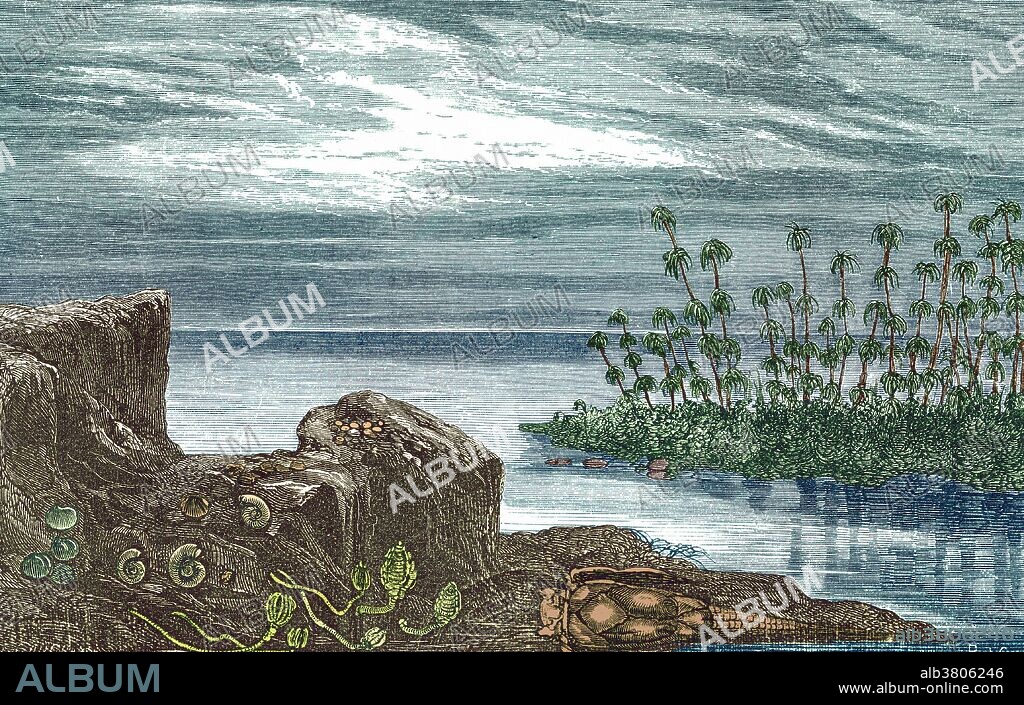The image is an advertisement for an album company, prominently featuring the URL "www.albumonline.com" and a contact number located in the bottom right corner. The word "ALBUM" is superimposed multiple times throughout the image in a semi-transparent, diagonal watermark, preventing reproduction. In the bottom left corner, there is a black box stretching across the entire bottom, containing the word "ALBUM" in gray text.

The depicted scene is calm and serene, with a large body of water that appears to be a lake or ocean, varying in shades of blue. The sky is gray and overcast with thick clouds, through which the sun faintly shines. In the foreground, to the left, a rocky landmass extends, varying in height and featuring green flora, including vines and tubular plants with curled-up ends. Among the rocks, small snails or worms are nestled, adding to the detailed nature landscape. In the middle right of the image, some snails are visible on the rocks, positioned near the water's edge.

Additionally, on the right side of the rocky foreground, there are tall, skinny palm trees rising from a piece of green land. An orange bug or similar creature is visible among the rocks. This detailed illustration merges elements of digital text and natural scenery, creating a composite that highlights the tranquil water scene and the dense, varied plant life.